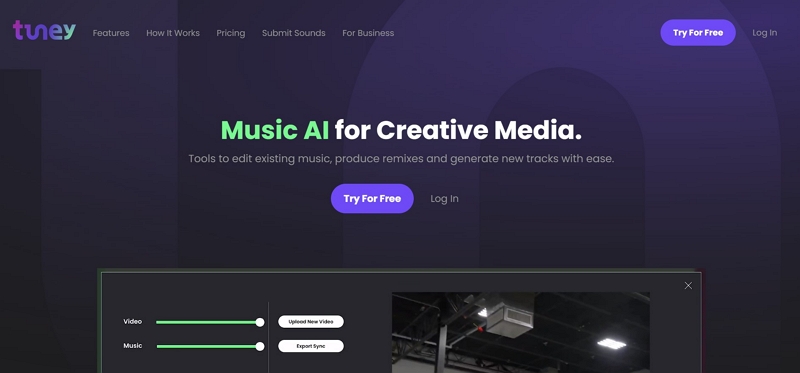The image shows a colorful screenshot of a website for a computer software called Toonie, displayed in landscape format. The Toonie logo is prominently featured, written in all lowercase letters. The 'u' blends seamlessly into the 'n', creating a worm-like appearance. The logo design transitions from purple on the left to blue in the middle, and finally to green on the right.

The website has a dark blue background that gives it a sleek and modern look. White text contrasts sharply against this background. At the top left of the screen are tabs labeled "Features," "How it Works," "Pricing," "Submit Sounds," and "For Business." On the right-hand side, there are options to "Login" or "Try for Free."

Dominating the center of the page is a large headline that reads, "Music AI for Creative Media." Directly beneath this headline, smaller subtext elaborates: "Tools to edit existing music, produce remixes, and generate new tracks with ease." Below this description, there's an ovular purple button with white text inviting users to "Try for Free," alongside a "Login" option.

Further down the page, there are toggle options for switching between video and music, though the exact functionality of these toggles is partially cut off in the image.